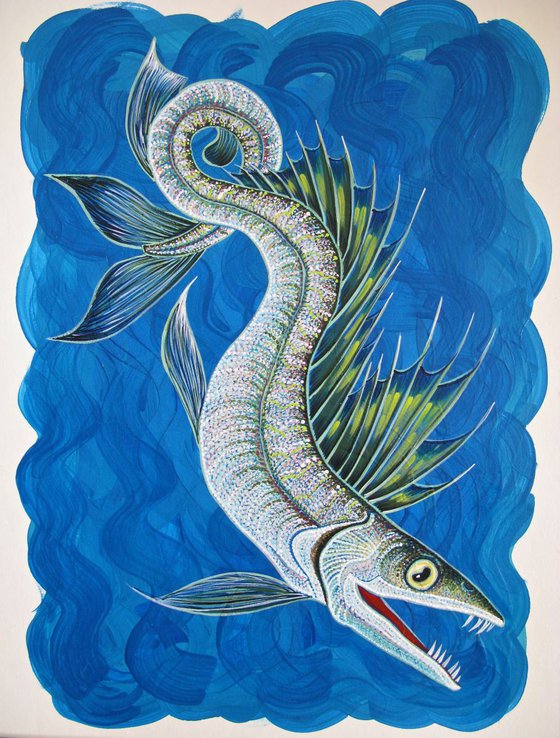The painting is rendered on a white, rectangular canvas. The background features a blue gradient, created with visible, vertical paint strokes that suggest the artist began at the top and pulled the brush downward. Central to the composition is a striking fish depicted in vivid green hues. The fish is oriented head-down towards the bottom of the canvas, showcasing its intricately detailed fins that blend shades of green, blue, and white. The tail fin, positioned towards the top, is highlighted with a lighter green tone. The fish's open mouth reveals a touch of red and a row of discernible teeth, adding a sense of dynamic realism to the artwork.